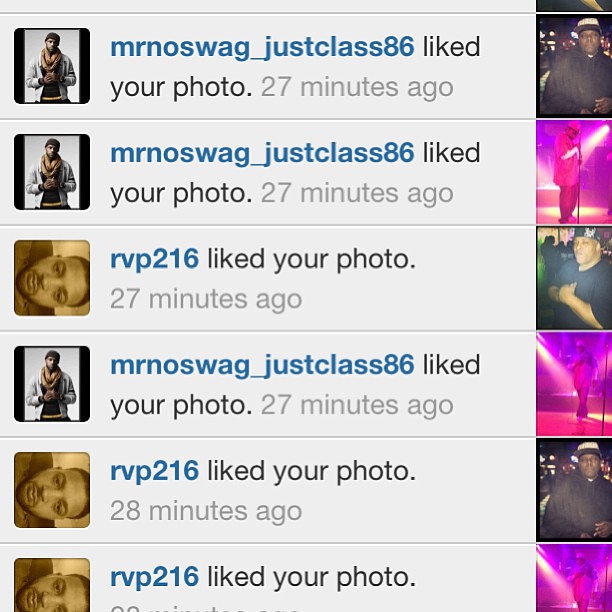The image is a screenshot capturing social media notifications of likes given to a photo. There are six distinct notifications arranged in rows, each displaying a thumbnail image on the left of the person who liked the photo and a larger image on the right showing the photo they interacted with. The text accompanying each notification indicates the users who liked the photo and the approximate time. 

Mr. No Swag, just class 86, is prominently featured, having liked the photo several times, specifically 27 minutes ago. Another user, RVP216, also liked the photo multiple times, with timestamps showing 27 and 28 minutes ago. The thumbnail images depict the users in posed photos, while the larger images on the right feature them in more casual, real-life settings, possibly in clubs or social gatherings. The overall background of the screenshot is light gray, with horizontal lines separating each notification, providing a clear and organized visual representation of the interactions received.